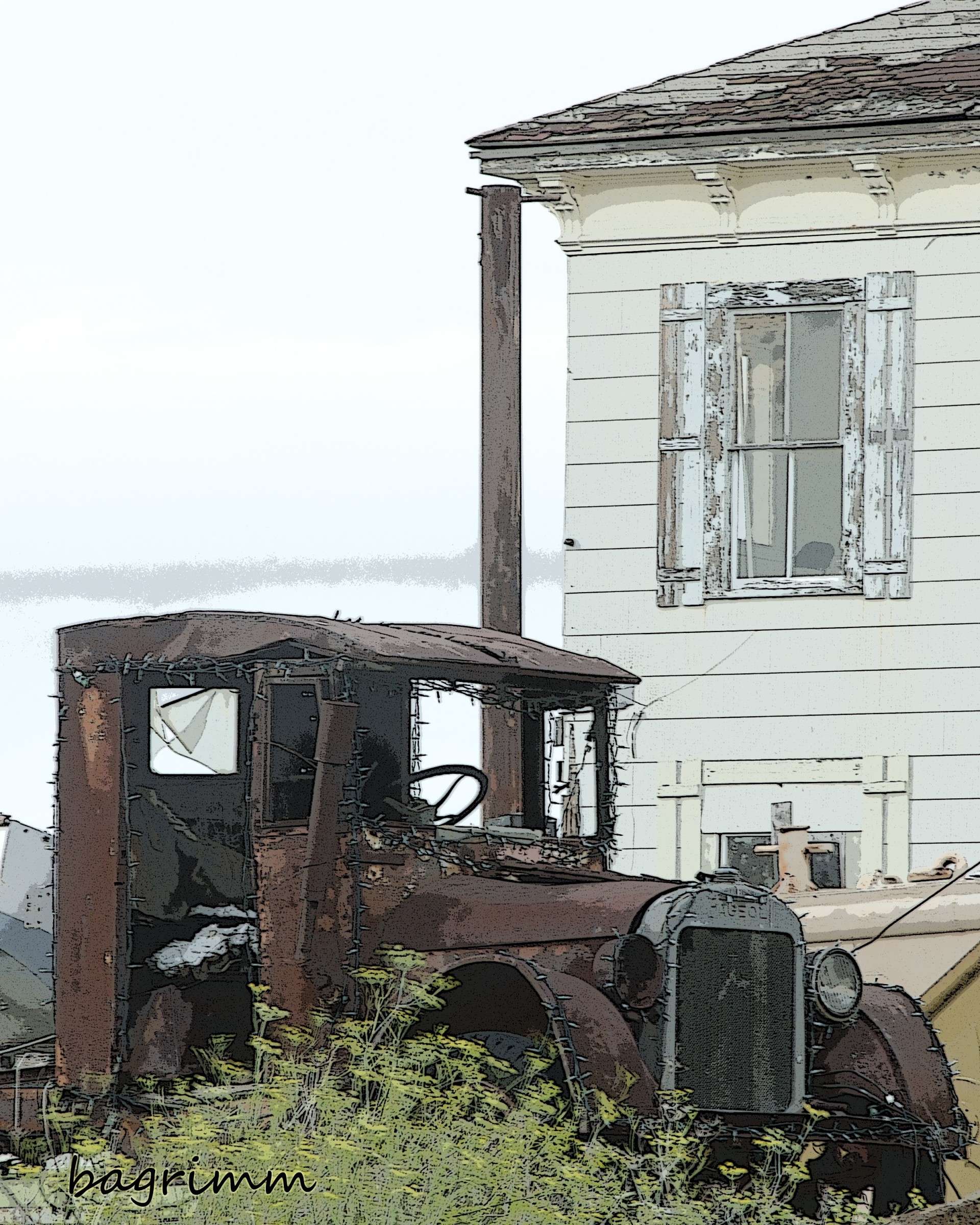The image depicts a digitally stylized drawing of an old, abandoned delivery truck from the 1940s, with a filter applied to enhance its outlined features, giving it a hand-drawn appearance. The truck, missing one headlight and full of rust, has broken and missing windows, and tall green grass grows around its deteriorated frame. Christmas lights are wrapped around various parts of the truck, including the windshield, doors, fenders, headlights, and grill, suggesting it might be used as a decorative piece. This truck is parked in front of a weathered, two-story white house with open, white shutters on its first and second-floor windows. There is a board supporting something to the left of the house, and a silver object behind the truck, which is unclear. The sky appears mostly clear with a gray streak from the middle to the left side. In the bottom left corner of the image, the artist’s name, "BAGRIMM," is visible in back letters. The color palette includes greens, browns, whites, yellows, and hints of blue and black, enhancing the sense of an aged, rustic scene.